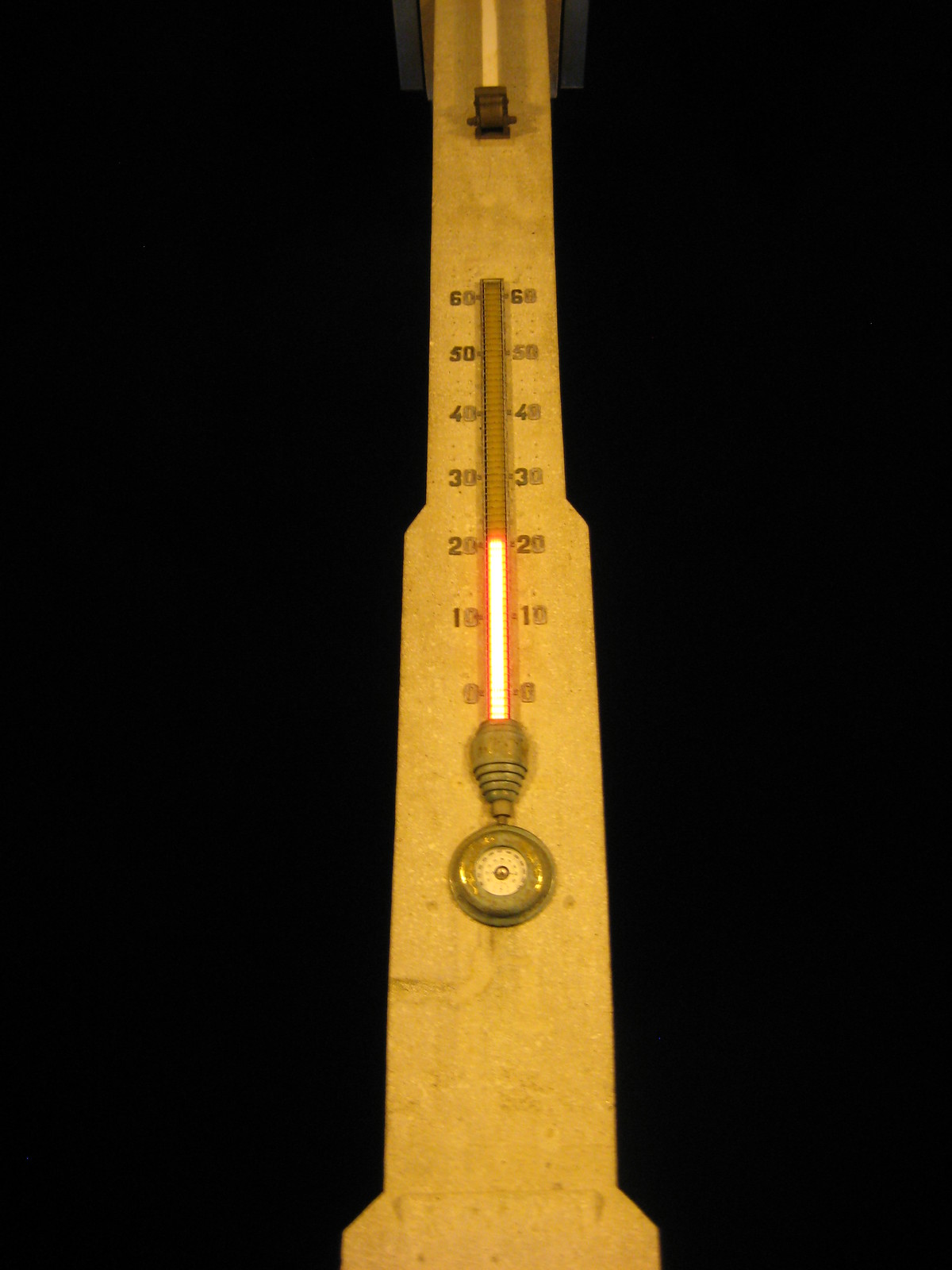This image showcases an antique metal thermometer set against a solid black background. The thermometer features a prominent rectangular gauge displaying various incremental lines within which mercury typically resides, although in this instance, there is a red line indicating a temperature of 20 degrees. The thermometer has a classic, old-time aesthetic, with the top section slightly narrower than the bottom, creating a subtle, symmetric taper. 

The functional part of the device, where temperature is indicated, occupies the central portion. The metal clasp at the base of the thermometer has a bronze hue with visible signs of rust, adding to its vintage appeal. The entire piece is well-crafted from a metallic material that appears slightly weathered, suggesting it has been well-used and aged over time. The image isolates the thermometer, highlighting its historical character against the stark contrast of the black background.